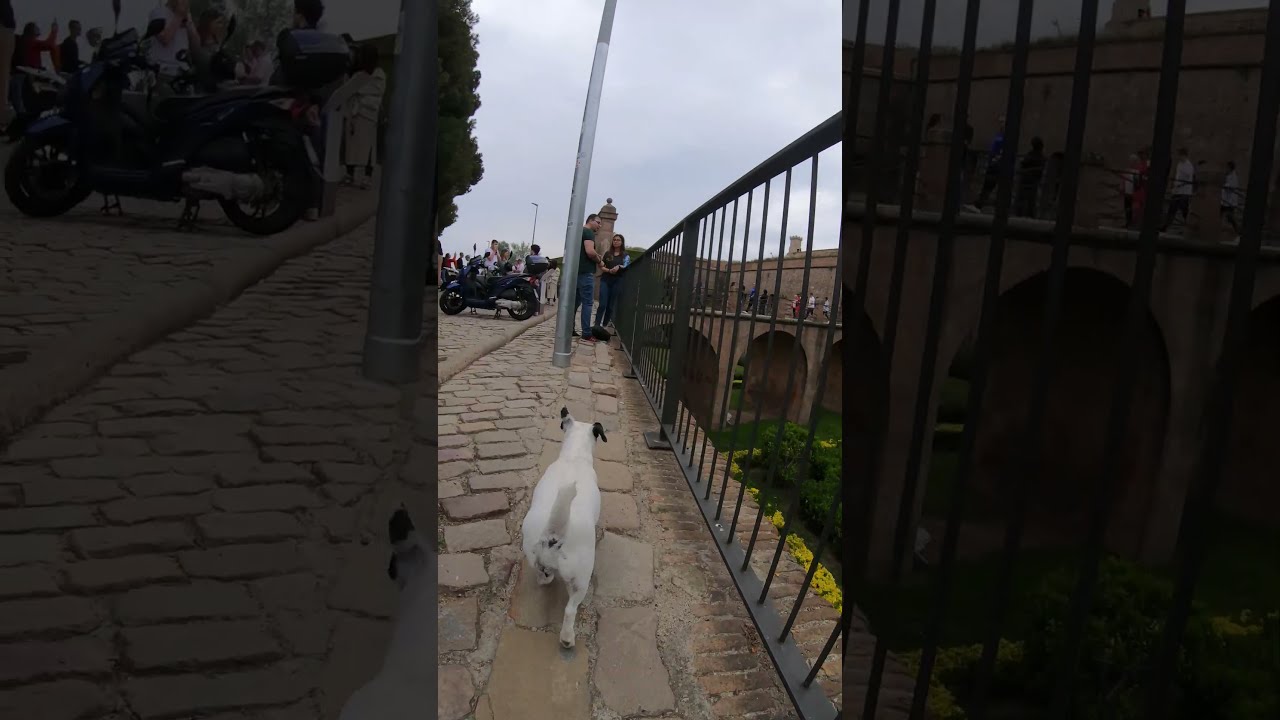The photograph captures a dynamic outdoor scene featuring a cobblestone sidewalk bordered by a black metal railing on the right. Dominating the foreground, a white dog with black ears walks towards a man and woman who are centered in the image. The man, in a green t-shirt and blue jeans, leans against a metal pole, while the woman in a blue top and blue jeans stands beside him, her back against the railing. A blue motorcycle is parked to the left of the couple, adding a pop of color to the scene. In the background, numerous people are dispersed, with some walking on what appears to be a bridge or elevated walkway. This structure overlooks a botanical garden teeming with vibrant yellow flowers and lush greenery. The upper portion of the image is dominated by a light blue sky, partially covered with clouds.